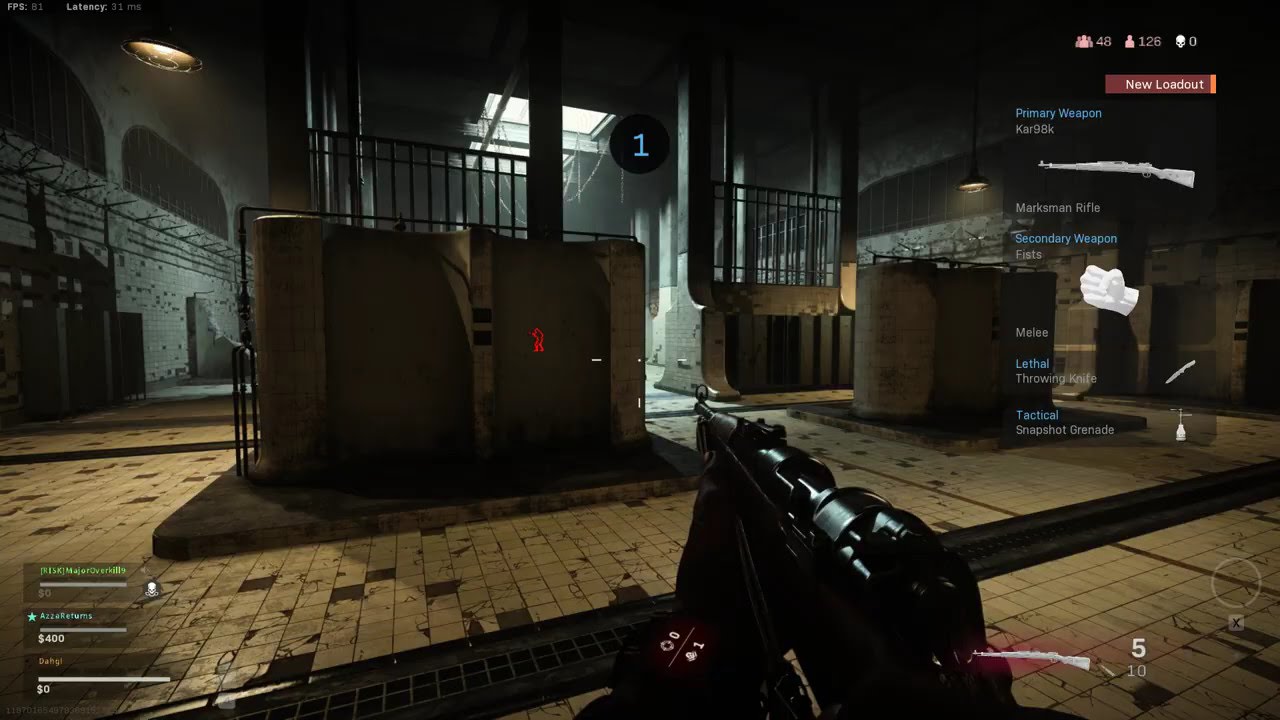This is a detailed screenshot from a three-dimensional shooter video game. The scene is set in what appears to be a dimly lit, extensive basement or industrial facility. Dominating the foreground is a rifle held by an unseen player, with the barrel slightly angled from the right side. The targeting reticle, comprised of a couple of dashes and a central dot, is centered on a red silhouette of a person, seemingly behind a wall.

The environment features worn-out yellow and brown tile flooring, some parts containing drainage grates. High up, an iron framework encloses this area, with cast iron fencing bars visible right in front. The grayish walls extend high into arched ceilings supported by heavy steel columns. Multiple barred windows enhance the prison-like ambiance. Toward the back, there's a prominent brightly-lit skylight or large light panel that contrasts with the shadowy surroundings.

On the right-hand side of the screen, a user interface displays detailed weapon information: the primary weapon, possibly a marksman rifle, and a fist icon indicating secondary options. Underneath these are sections labeled lethal and tactical. Additionally, a display towards the bottom corner shows the player's available money, which stands at $400 for in-game purchases.

Scattered vats on the floor suggest an industrial or manufacturing scenario. Red letters are visible vertically on one of the vats, although their exact meaning remains unclear. The entire scene depicts a tense and atmospheric location, fitting for a tactical engagement in this video game.